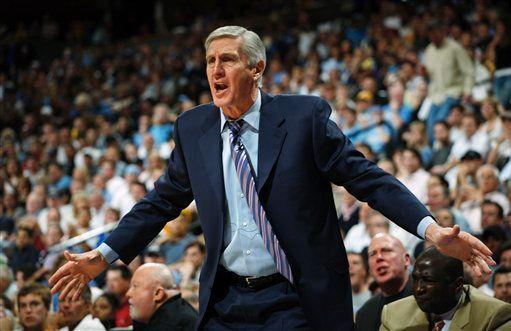In this detailed, color photograph, a gray-haired man stands at the dead center, angrily shouting towards something off-screen to the left. His arms are extended straight out at waist level, with fingers outstretched, embodying a gesture of frustration or command. He is dressed sharply in blue dress pants secured by a black leather belt with a silver squared buckle, a matching blue sports coat, a light blue button-up collar shirt, and a blue, silver, and purple striped tie.

Behind him, the scene unfolds in a stadium or arena setting, where multiple tiers of audience members fill the stands, their attention also directed leftward toward the off-screen commotion. The backdrop showcases thousands or perhaps hundreds of spectators, save for one individual visible making his way down the steps towards his seat, further emphasizing the collective focus. The photograph captures a moment of intense emotion amid the sea of attentive onlookers.